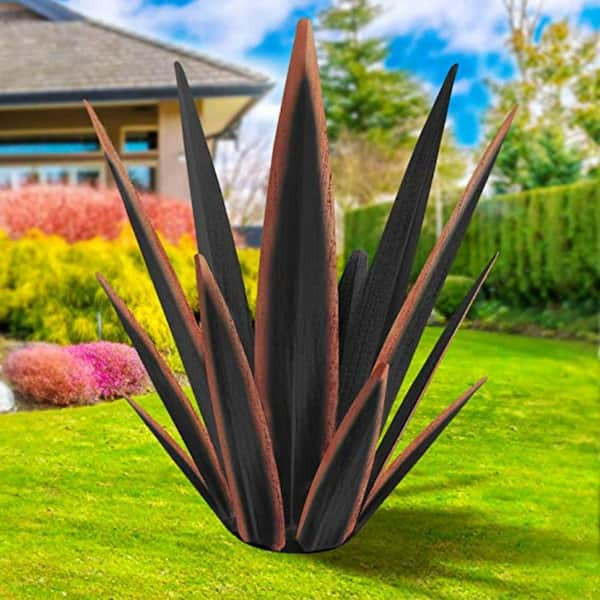The image appears to be AI-generated, featuring a large, spiky plant resembling an agave or possibly a fern, prominently centered on a lush green lawn. The plant has striking dark brown or dark green leaves with lighter brown or orangish-red edges, giving it a sharp, imposing appearance. It seems to be unnaturally placed, as if it is merely sitting atop the ground rather than growing from it. In the background, a house with a tan roof and individual shingles is visible, complemented by reflections of blue sky and clouds in the windows. Surrounding the house are various bushes, including a pink bush, a yellowish-green bush, and a reddish bush. On the right side, there is a hedge with trees, set against a backdrop of blue sky with scattered clouds. Overall, the image's symmetry and certain elements suggest it may have been manipulated or created through digital means.